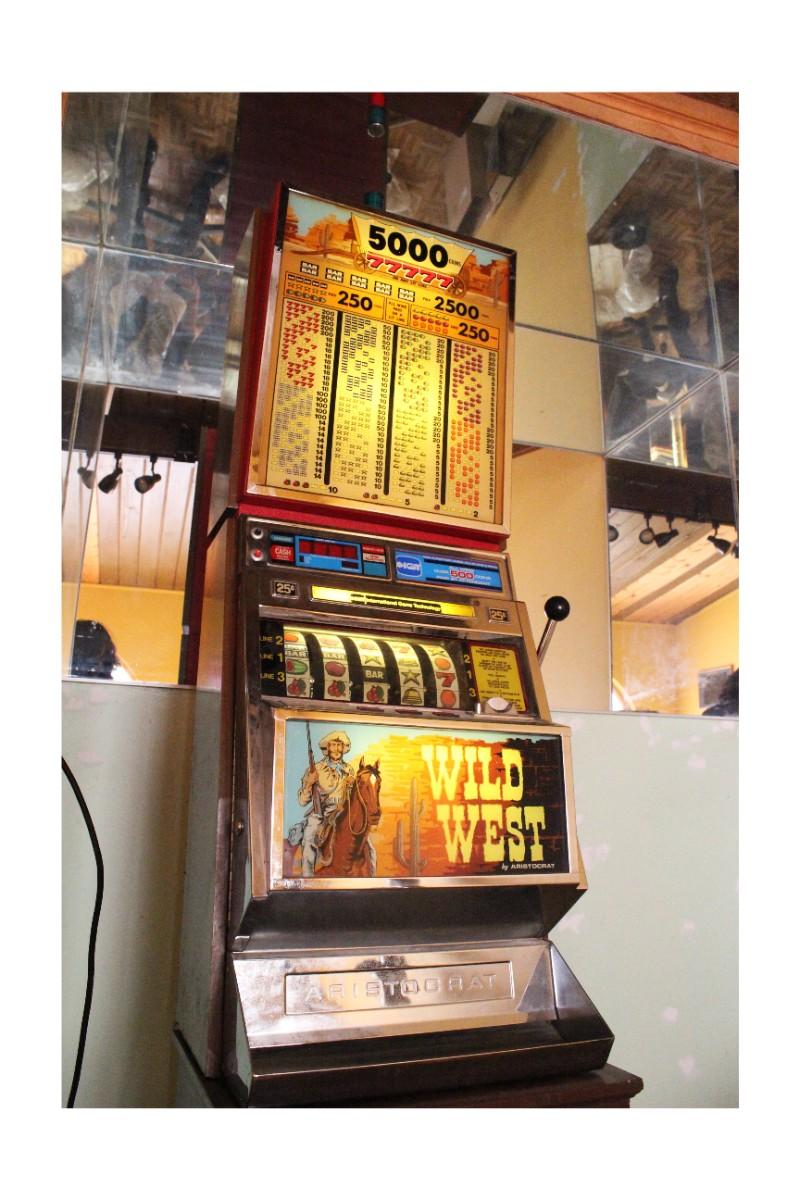This photograph captures an old-style slot machine from the Wild West series, likely dating back 30-40 years. The machine exhibits a vibrant color scheme of yellows, oranges, and browns, evocative of a desert or Western theme. Dominating the front of the machine is the Wild West logo in yellow font, accompanied by a vivid depiction of a cowboy dressed in tan riding a bronze horse, with a green cactus also featured in the image. At the top of the machine is a detailed payout legend, providing information on the payout for different combinations. The slot machine includes a lever on its right side and a payout tray at the bottom for collecting coins. The backdrop of the photograph features a white wall partially obscured by a row of mirrored tiles, with lighting from the ceiling casting a soft glow into an alcove. The setting suggests the machine is placed against a wall, with various stored items visible behind the glass structure in the background. The overall scene is not cartoon-like but rather a realistic snapshot, emphasizing the vibrant and nostalgic details of the slot machine.